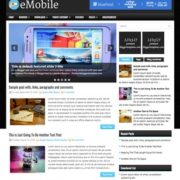A highly pixelated and blurry screenshot, presumably taken from a mobile phone, dominates the image. The screenshot appears to be square-shaped and seems to capture what might be a webpage or an application interface related to "e-mobile." In the upper left corner, the text "e-mobile" is faintly visible. A distinctive blue stripe stretches from the upper center to the upper right of the image, though the content within this stripe remains indistinguishable due to the blurriness. 

Beneath the blue stripe, a series of seven tabs with faint white font can be seen, providing minimal guidance on the page's navigational structure. Below these tabs, there might be an image of a phone displayed horizontally, although the lack of clarity makes this uncertain. Further down, the layout suggests the presence of news articles, a possible picture of a living room, and multiple light blue buttons whose labels are unreadable.

On the right side, there’s a vertical alignment of various elements: two black squares at the top, followed by a blue button, then two additional black squares. This column continues downward, featuring what appear to be three articles, interspersed with black stripes containing writing, though none of the text is legible. This screenshot, likely of an e-mobile news page or similar interface, is too small and blurred to provide detailed information or clear readability.